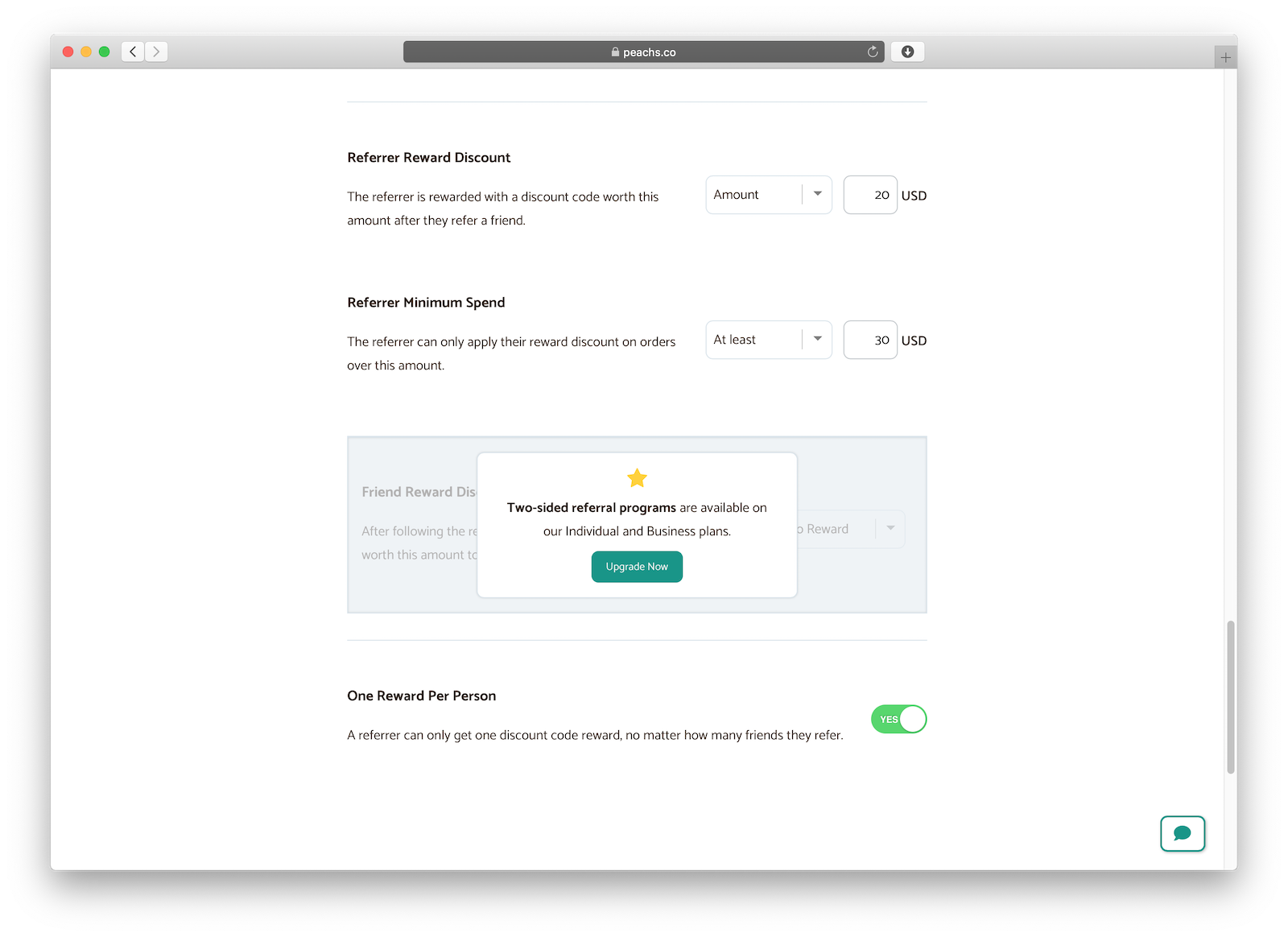A screenshot of the website "peaches.co" with a slightly blurry URL at the top. The first section is titled "Referral Reward Discount." This section explains that users receive a discount code worth $20 when they refer a friend. To the right, there's a label "Amount" with "20 USD" displayed next to it. Below, another section titled "Minimum Spend Requirement" indicates that the reward discount can be applied only to orders over $30. To the right, it states "at least 30 USD." 

A highlighted box with a star at the top contains the text: "Signup for our referral program available on our individual and business plans." Below, a prominent green button labeled "Upgrade Now" is visible. At the bottom of this section, there's a note that says "One reward per person: A referrer can only get one discount code reward no matter how many friends they refer," with a toggle button switched on, displaying "Yes."